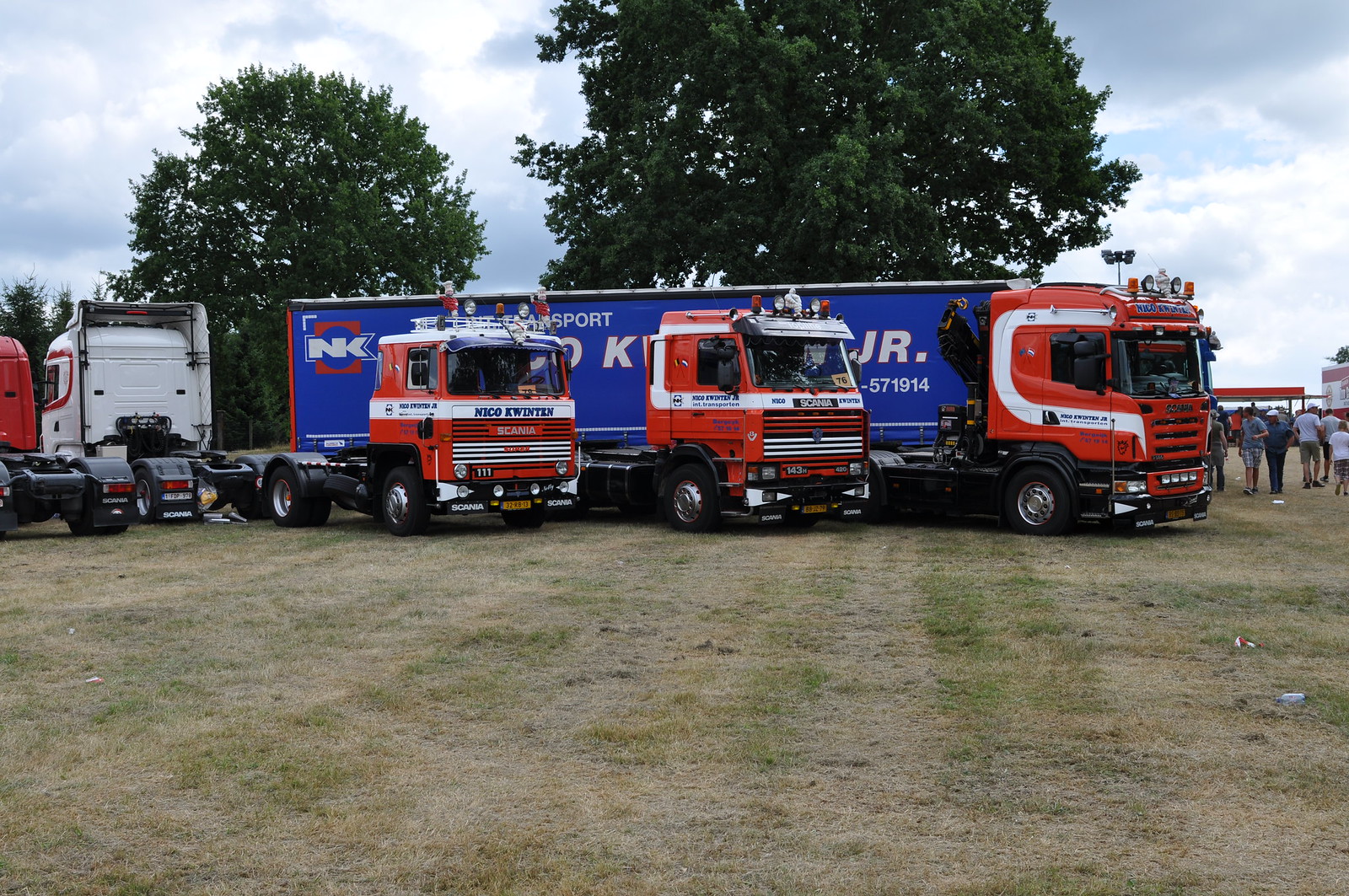This photograph captures a gathering of semi-trucks parked on a grassy field that appears trampled and worn. The trucks, primarily from the brand Scania, are situated centrally from right to left in the image, with their vibrant red and white cabs drawing the eye. Amongst them, there are three red trucks and one white truck; a partial view of a fourth red truck can also be seen. Notably, none of these trucks have their cargo beds attached, except for one truck featuring a large blue shipping container with white writing that includes the letters "NK" and some transport-related text. This container is located behind the other trucks. The scene buzzes with activity as several people walk along the side of the truck with the blue trailer, most of them facing away. The trucks, similar in design, are mostly aligned in the same forward-facing direction, except for the white and adjacent red truck, which face the opposite way. This snapshot, likely taken at an event or park, encapsulates both the sturdy, industrial presence of these vehicles and the casual human interaction around them.